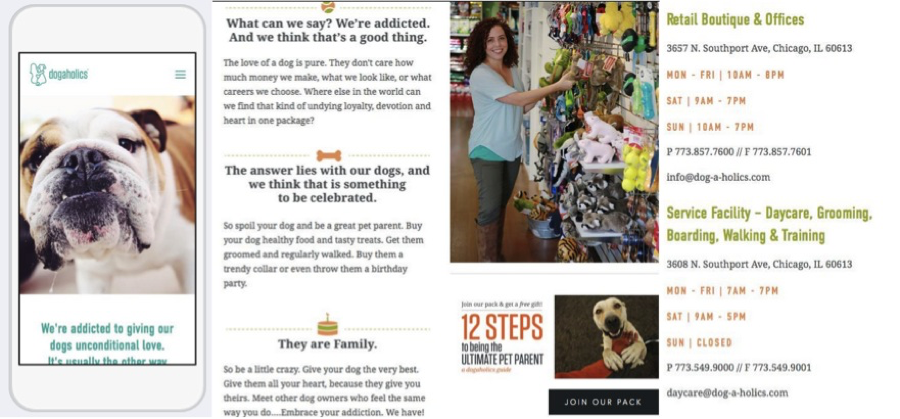The image features an adorable pug positioned to the left, exuding charm with its curious expression. At the top of the image, the bold text reads "Dogaholics," celebrating the deep bond between dogs and their owners. The accompanying text conveys a heartfelt message: "We are addicted to giving our dogs unconditional love. It's usually the other way around. We are addicted, and we think that's a good thing. The love of a dog is pure; they don't care about our earnings, looks, or careers. Where else can we find such undying loyalty, devotion, and heart in one package? The answer lies with our dogs, and that's something to be celebrated. They are family. So go ahead, be a little crazy. Give your dog the very best, all your heart because they give you theirs. Meet other dog lovers who feel the same way. Embrace your addiction." This description captures the essence of the unique and profound connection shared between dogs and their human companions.